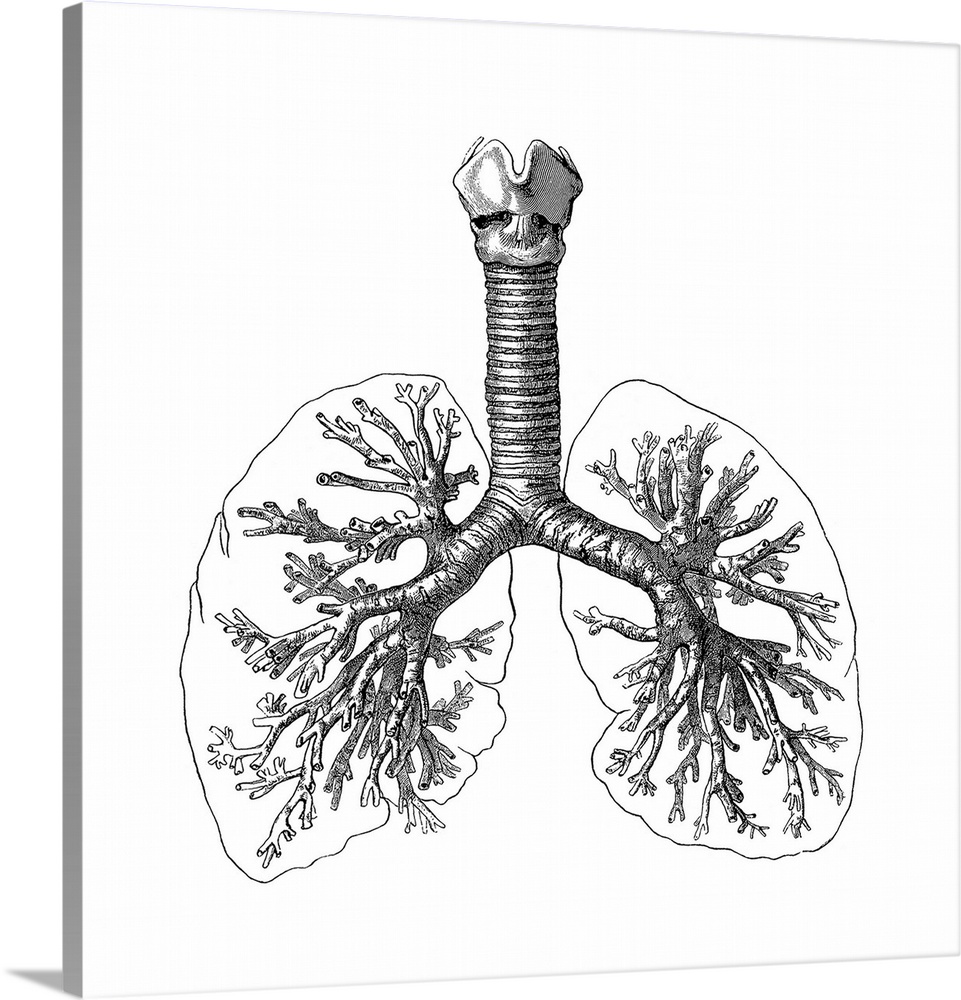In this black and white, pencil-drawn image, an artist has intricately rendered the human respiratory system, specifically emphasizing the lungs and their branching structures, invoking the visual metaphor of tree branches. The image prominently features the windpipe extending into the upper airway, which gracefully diverges into two main sections, each representing a lung. These branches, reminiscent of a tree's network of limbs, symbolize the intricate bronchial tubes. At the top of the diagram, the bone structure is distinctively shaped like a crown, lending an almost regally anatomical aspect to the depiction. The image's animated style is highlighted by its placement on a thick, poster board-like medium, which adds depth and a touch of gray to its overall presentation. The upper portion of the drawing also alludes to the throat and possibly the chin area, completing the detailed anatomical illustration that blends both biological accuracy and artistic elegance.